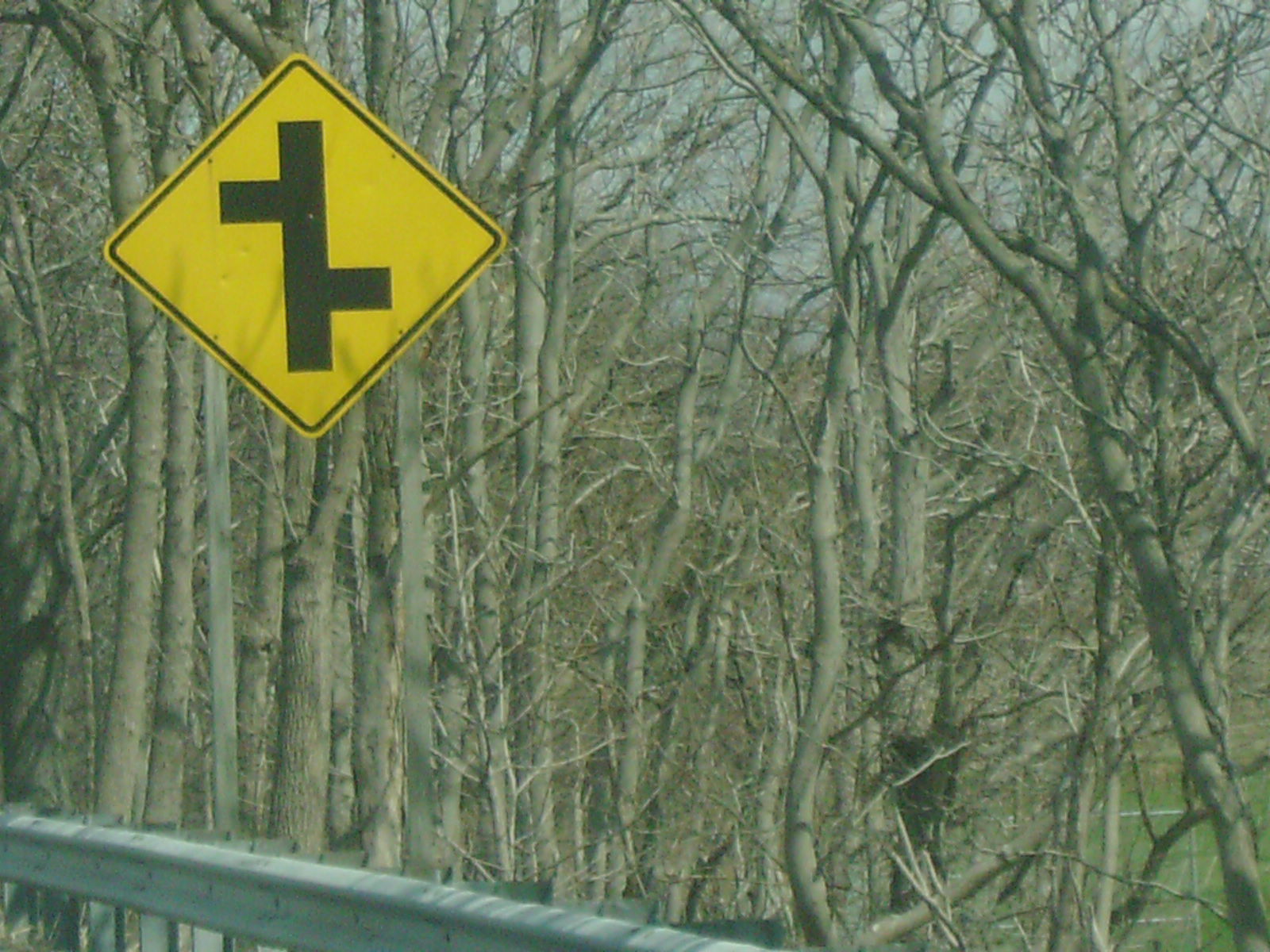This outdoor photograph, likely taken during a cold winter month, captures a stark, leafless landscape dominated by a cluster of thin, barren trees with crooked branches twisting in various directions. Centrally on the right, a prominent tree curves distinctly to the left before straightening and extending upwards. A silver guardrail with tall, rectangular legs runs across the lower left of the image, featuring several bolts and darker dots down its center. Connected to the guardrail is a gray post supporting a yellow, diamond-shaped street sign bordered in black. The sign displays a black vertical line intersected by two horizontal black lines on the left and right, likely indicating a road intersection.